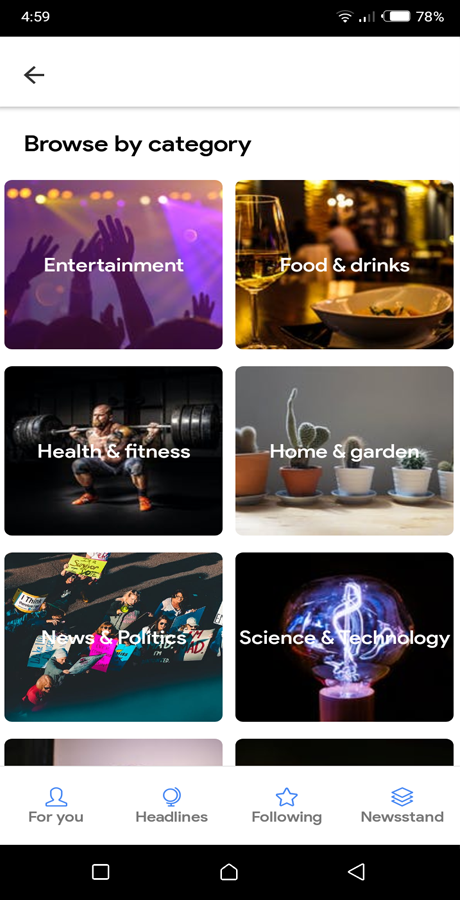This is a screenshot captured from a cell phone. The background of the image is predominantly white. At the top of the screen, a black status bar displays the time in the top left corner while the top right corner shows the Wi-Fi signal, cellular signal strength, battery icon, and battery percentage, all in white against a black background. 

Below this, there is a user interface element with a left-facing arrow on the left, which likely indicates a way to navigate back to the previous menu. Underneath this, a grey line separates the arrow from a bold, black heading that reads "Browse by Category." 

The main section of the image features six thumbnails arranged in a grid, each representing a different category:
1. The top left thumbnail shows a vibrant nightclub or concert scene bathed in purple light with hands raised in the air. It is labeled "Entertainment."
2. To the right, another thumbnail showcases a table set with food, drinks, and candlelight, labeled "Food & Drinks."
3. The middle row on the left has an image of someone lifting heavy weights at a gym, labeled "Health & Fitness."
4. To the right in the middle row, a thumbnail displays four cacti in pots, labeled "Home & Garden."
5. The bottom row on the left shows an image labeled "News & Politics" that includes several people.
6. The bottom row on the right has a light bulb icon, labeled "Science & Technology."

Additionally, you can see the tops of two more thumbnails at the bottom of the screen, though their contents are not visible.

At the bottom of the image is a navigation menu bar. It features four options: "For You" with an outline of a person's head, "Headlines" denoted by a headline icon, "Following" represented by a star, and "Newsfeed" shown with a pile of paper icon. The very bottom of the screen shows a black bar containing a white square on the left, a home symbol in the center, and a left-facing arrow made of a triangle on the right.